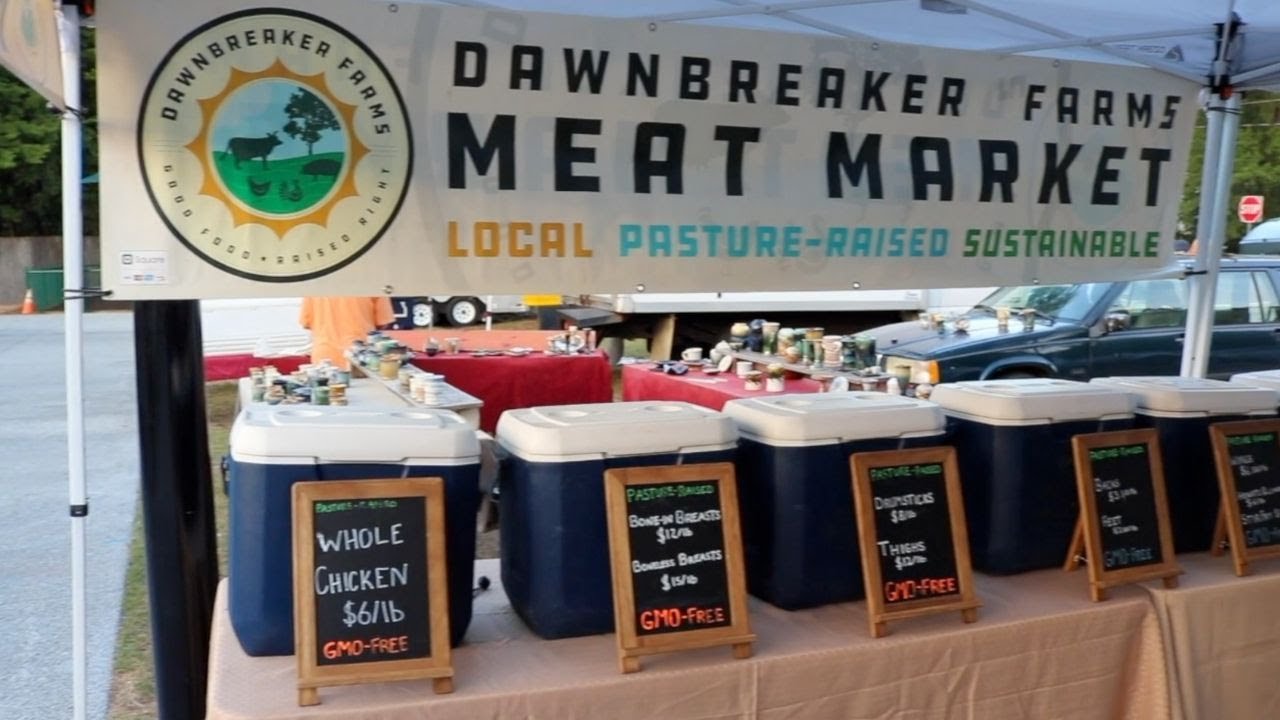This image depicts an outdoor meat market stall belonging to Dawn Breaker Farms. The prominent sign above the stall reads "Dawn Breaker Farms Meat Market," with the farm's logo on the left side, featuring a pastoral scene with a cow, chickens, a pig, a tree, and a yellow sun against a blue sky and green grass background. Beneath the farm name, the sign emphasizes the farm's commitment to being "Local, Pasture Raised, Sustainable." 

In the foreground of the image, there are several tables, including one with a pink tablecloth laden with dark blue coolers that have white tops. Each cooler is accompanied by a small chalkboard sign detailing its contents and prices: Whole Chicken at $6 per pound, Boneless Breast at $15 per pound, Bone-in Breast at $12 per pound, Drumsticks at $8 per pound, and Thighs at $12 per pound, all highlighted as GMO-free.

Further back, there are additional tables covered in red tablecloths displaying various products. Visible behind these tables are a blue station wagon, trailers, a stop sign, and some people approaching the stall. One man in an orange shirt can be seen attending to the market setup.